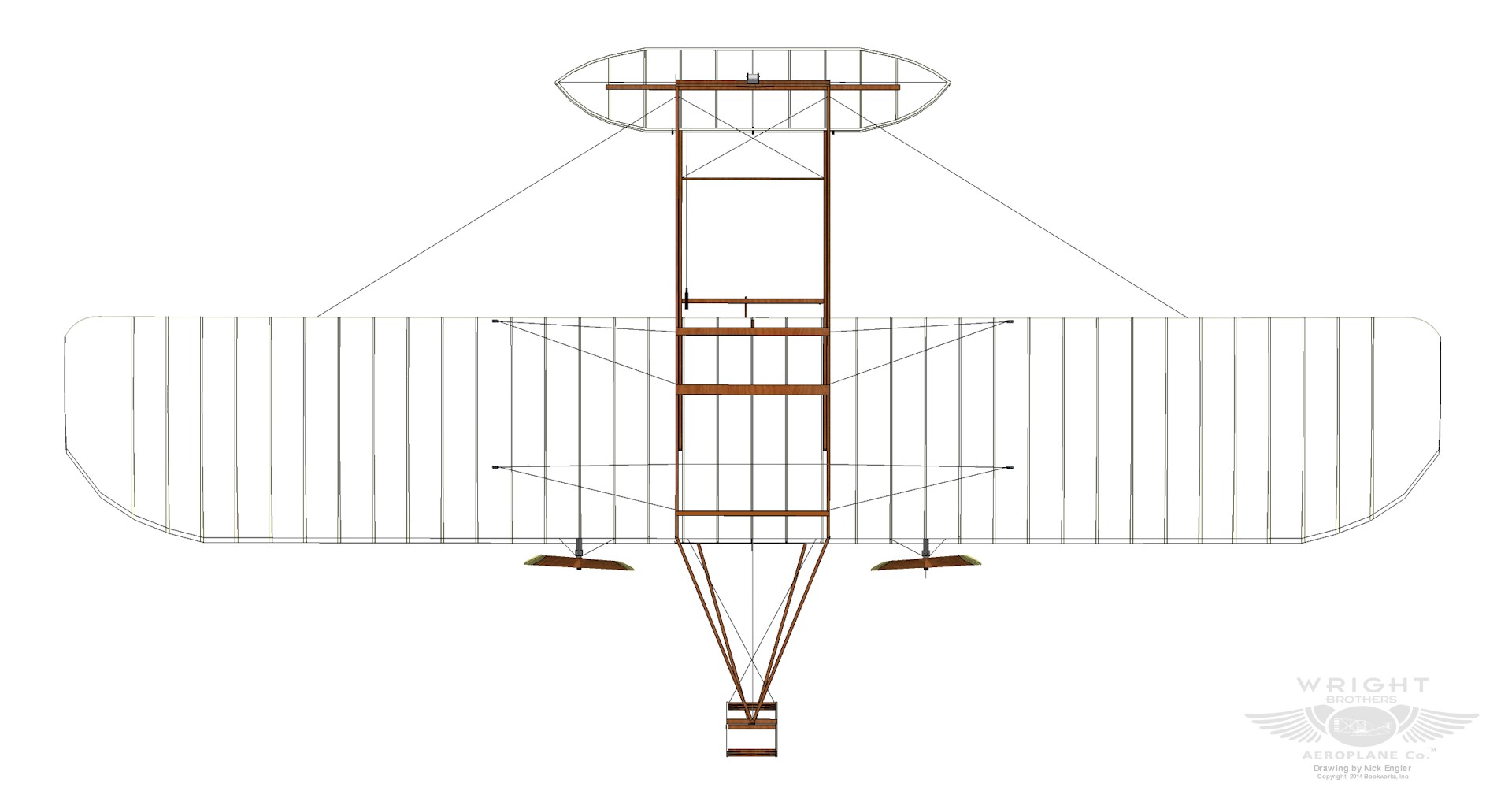This image is a detailed top-down diagram of an old-fashioned airplane, reminiscent of the Wright Brothers' design. The airplane is illustrated with a combination of black lines and brown accents, indicative of wooden components, set against a white background. The aircraft features a prominent cone-shaped nose and is equipped with two propellers located on either side of the cockpit area. The main wing, notably large, stretches across the center of the plane, while a smaller wing is positioned at the tail. The drawing bears a watermark in the bottom right-hand corner that reads "Wright" above a small oval with bird wings extending from it, also containing the words "Aeroplane Co." Though some of the text is hard to discern, this watermark adds to the historical authenticity of the blueprint-like image.